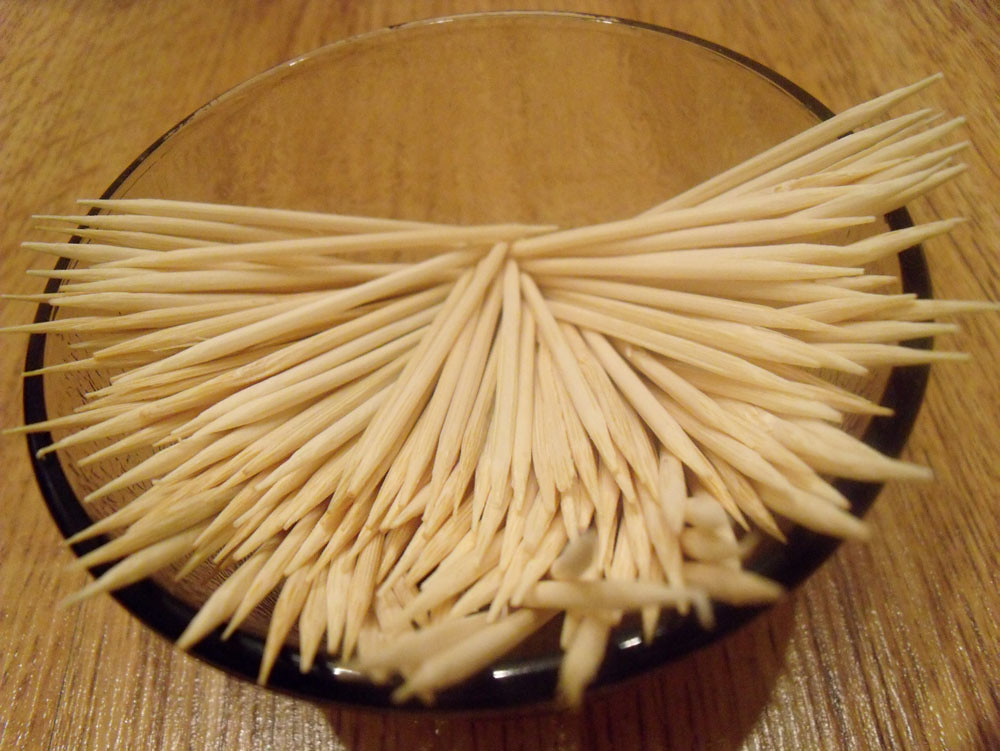The image is a close-up, low-angle photograph of a clear round glass container holding dozens of wooden toothpicks. The container's thick rim, which appears dark and almost black in some parts, frames the scene. Inside the container, the toothpicks are arranged with one end tightly clustered in the center and the other ends fanning out, with many of them protruding over the rim. The glass bowl sits on a wooden table with a prominent grain running upward in the image. The texture of the table adds to the rustic feel, and the container casts a small shadow. No other elements are present in the photograph, keeping the focus on the detailed arrangement of the toothpicks within the glass bowl.